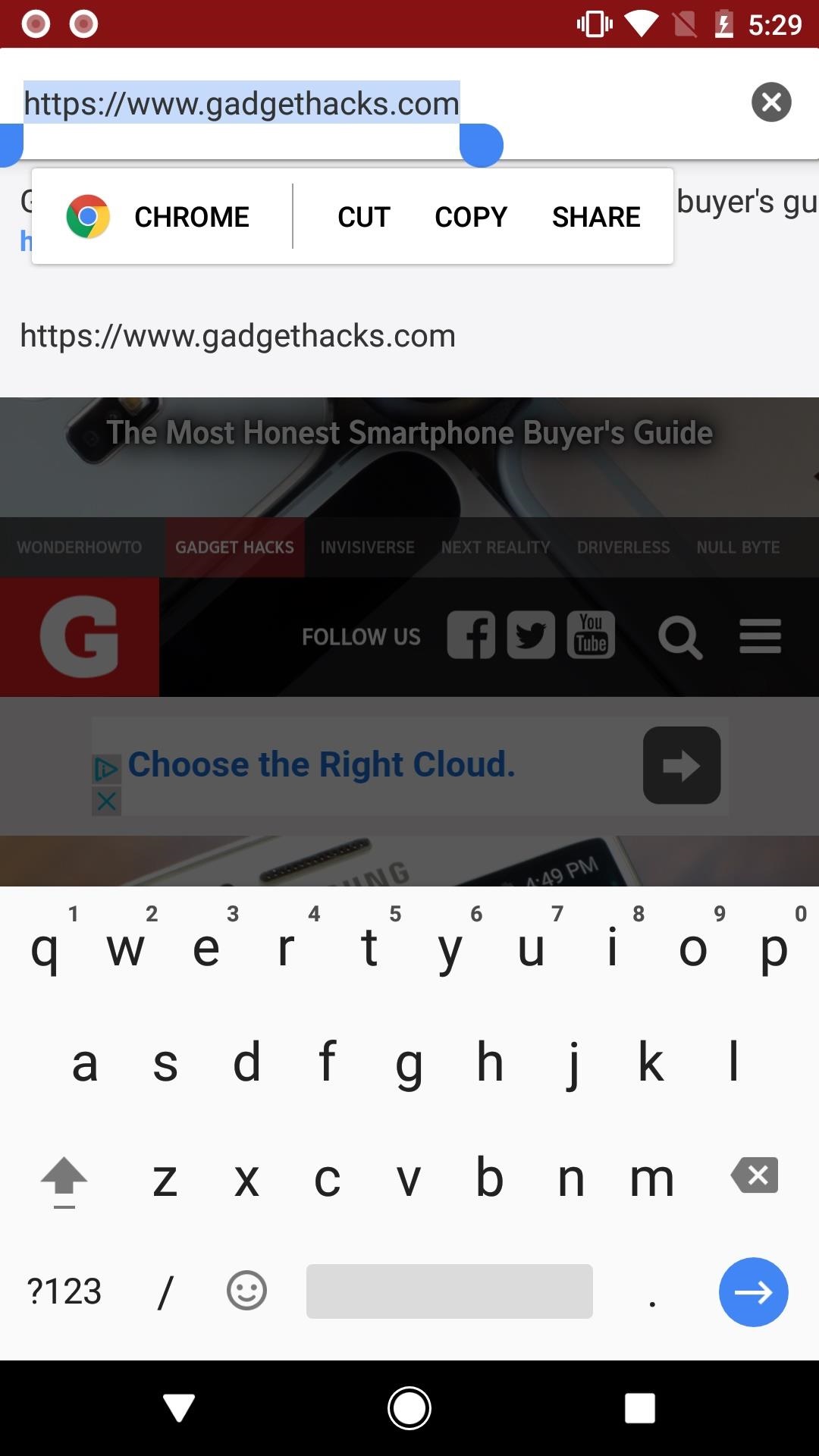A highly detailed screenshot of a smartphone screen with numerous visible elements: 

At the top, a thin reddish-brown bar spans the width of the screen. In the top-left corner, there are two small white circles, while the top-right corner displays several white icons, including a cell phone, Wi-Fi symbol, an icon resembling a piece of paper with a line through it, and a battery indicator showing minimal charge and a lightning bolt within. The time reads "5:29" in the top-right corner. 

Beneath this are two highlighted elements: a URL "https://www.gadgethacks.com" highlighted in blue to the left, and a gray circle containing a white "X" to the right. 

Further down, a pop-up bar features the Chrome logo to the left, followed by the text "Chrome," and options for "Cut," "Copy," and "Share" are aligned to the right. The pop-up partially obscures the underlying webpage, which is slightly grayed out. 

The visible part of the webpage shows the URL again in black text and a partially visible image containing the title "The Most Honest Smartphone Buyer's Guide." 

Directly below this web content, the smartphone's virtual keyboard appears on a white background, showing a QWERTY layout, and at the very bottom of the screen, a black horizontal bar features a white down arrow, a white circle, and a white square, aligned from left to right.